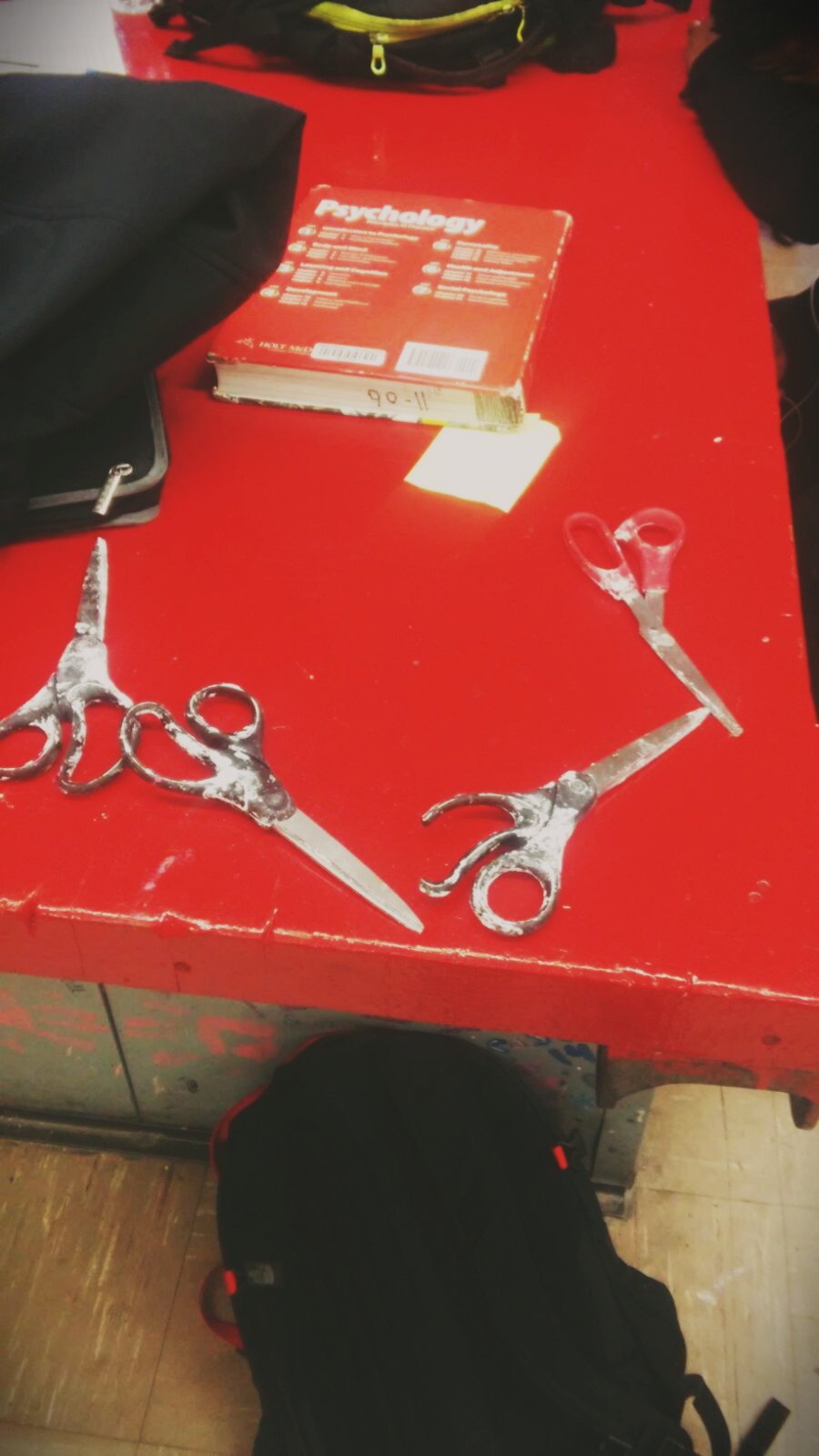In this photograph, we see a spacious red workbench with a painted metal surface. The bench appears to be in a classroom or workshop environment, and resting on it are four pairs of shiny, stainless steel scissors—one of which has a broken handle. A red book titled "Psychology" lies face down on the bench, with its title and sections visible on the cover. Adjacent to the book are two bags: one completely black and the other black with a yellow zipper. Below the bench, there's a sturdy steel base, with a black backpack leaning against it, noted for its distinctive red trim. The floor beneath the bench is composed of light brown vinyl tiles featuring subtle red streaks. The photograph captures a sense of an academic or creative workspace, cluttered with learning materials and personal belongings.